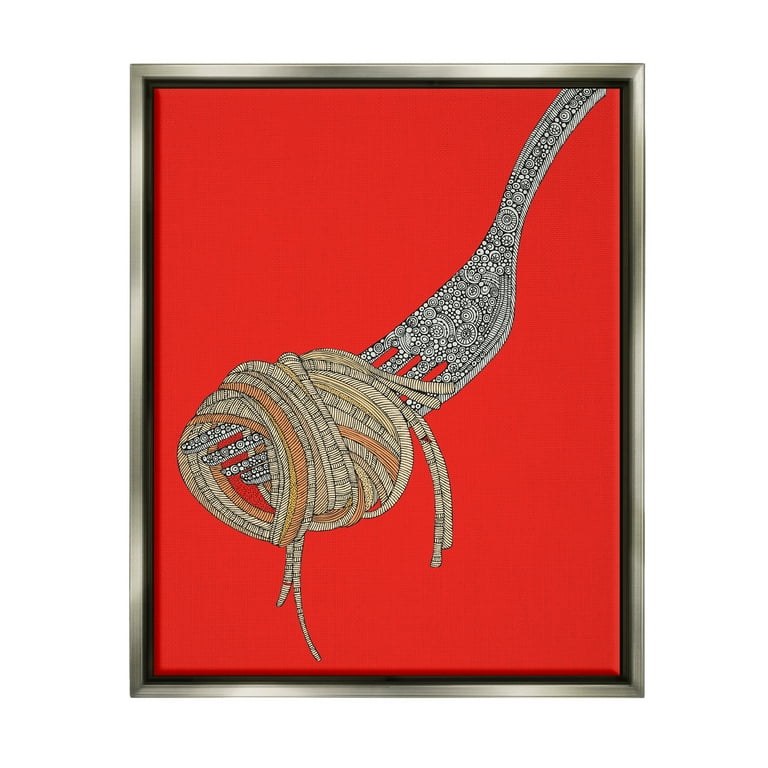This captivating artwork features a silver fork, intricately adorned with geometric and swirling patterns, diagonally extending from the upper right corner down towards the center of the canvas, against a bold, eye-catching muted red background. Wrapped around the fork are twirls of spaghetti, depicted in various shades of brown and yellow, resembling textured yarn. The noodles cascade towards the bottom of the artwork in a loose, abstract manner. This rectangular piece is enclosed within a silver frame, which includes a small black edge on the inside, lending it a polished and gallery-worthy appearance. The overall composition, marked by its vivid colors and intricate detailing, stands out as a striking example of contemporary art.